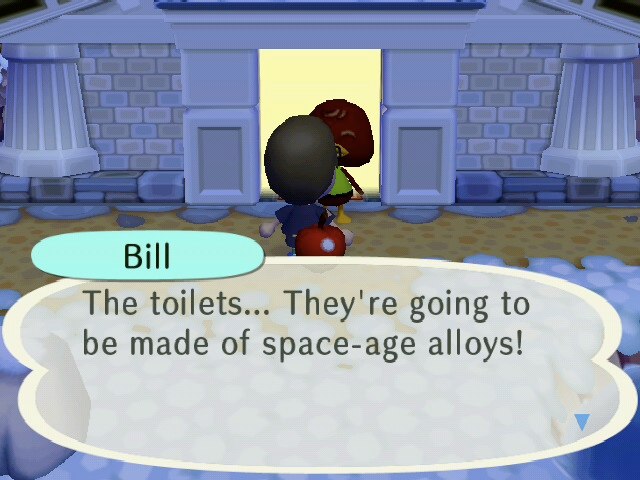The image appears to be a low-resolution, animated screenshot from a mobile role-playing video game. It depicts a conversation between two cartoonish characters with exaggerated features. The male character, identified by the green-shaded circle as "Bill," has gray hair and a big head, wears a blue shirt and shorts, and lacks detailed fingers. He is positioned with his back towards the viewer, standing near a red apple. The female character, partially visible, faces Bill and wears a green tank top and possibly a skirt. They are both situated in front of a building with blue walls and an open doorway, suggesting an indoor setting. Below the characters, a large, light purple dialogue bubble with a blue arrow contains text stating, "The toilets... they're going to be made of space age alloys!" The overall graphic quality is poor and pixelated, reminiscent of basic mobile phone games.